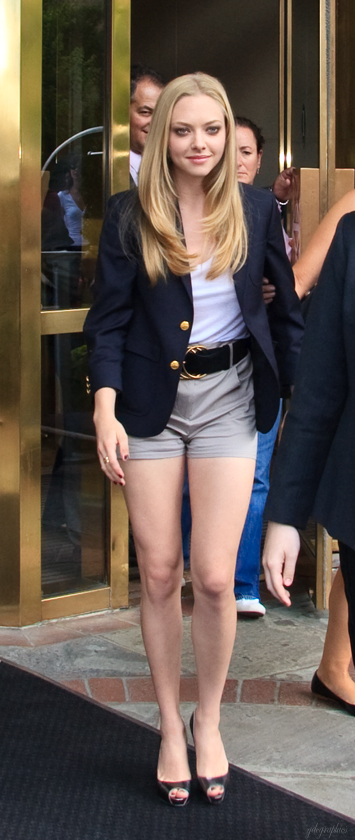In this detailed photograph, a young woman, who bears a striking resemblance to actress Amanda Seyfried, stands prominently in the center. She is decked out in a stylish ensemble featuring extremely short gray shorts secured with a large black belt adorned with three black buckles. She pairs this with open-toe black high heels, revealing her painted toenails. Her upper attire includes a silky white tank top layered with a tailored blue business coat, fastened with two gold buttons. The woman's long, layered blonde hair cascades down, framing her face as she looks ahead with a subtle smile. She appears to be outside, possibly exiting a hotel, as suggested by the gold metal framing a clear windowed doorway and the black rug transitioning to a cement pavement area. Though other people are in the vicinity, they are mostly obscured, with only the leg of another woman, who holds onto her arm, visible. The overall scene suggests a polished, public moment, capturing the essence of her poised and fashionable appearance.